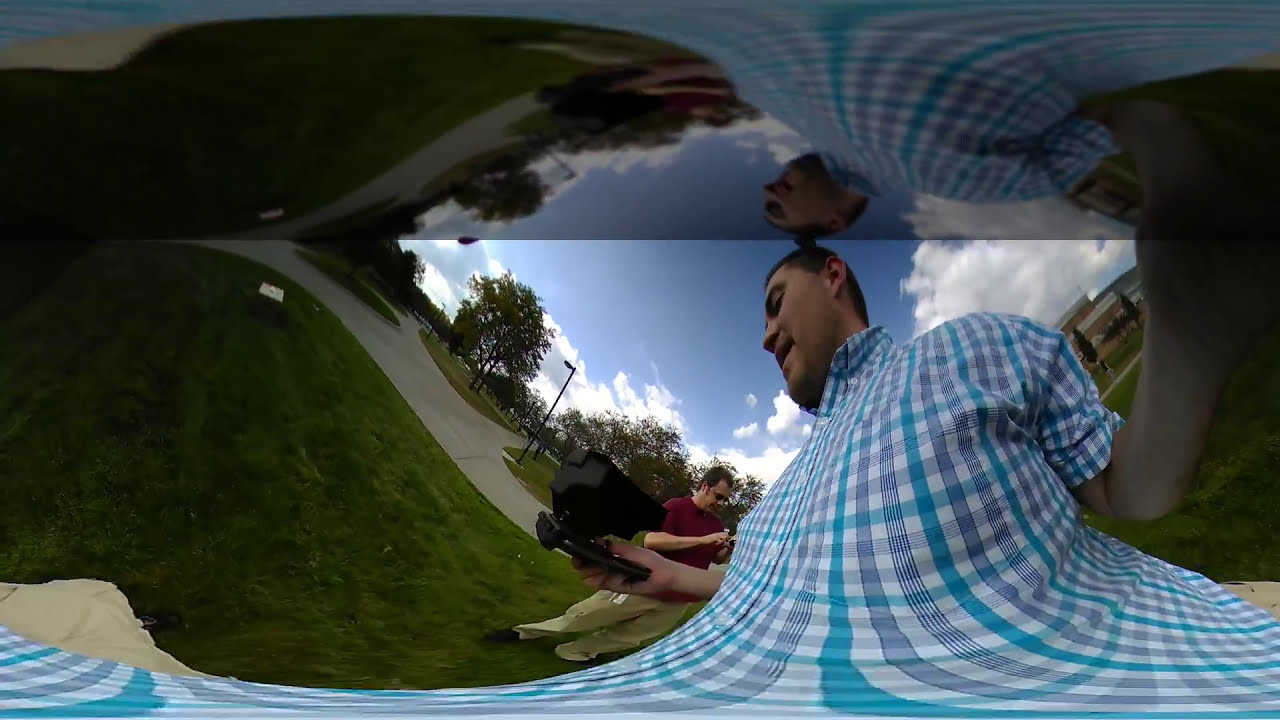The image captures a slightly distorted, panoramic view, possibly from a doorbell camera, featuring a Caucasian male holding a black camera in his right hand. He is wearing a collared, button-up shirt with blue and white stripes forming a hatched pattern. His short dark hair is neatly cut, and he is relatively clean-shaven. The man is looking down at the camera while standing on a cement area. In the background, another Caucasian male can be seen wearing a red short-sleeve t-shirt and beige pants, standing on a grassy lawn with a sidewalk beside him. The scene is set in what appears to be a park, with several walking paths, green trees, a light pole, and a blue sky dotted with white clouds.